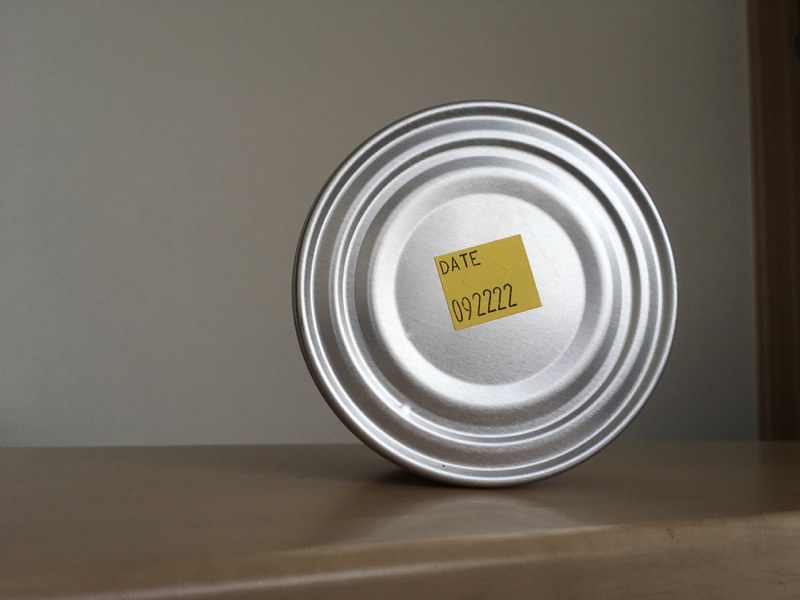On a glossy, light brown wooden countertop or shelf, an aluminum can lays on its side, its circular end facing the viewer. The reflective surface of the can catches the surrounding light, highlighting its sleek metallic design. The can is adorned with a yellow sticker in its center, which reads "DATE" followed by "09-22-22," presumably indicating its expiration date. The backdrop features a gray-colored wall, complemented by a light brown trim that likely outlines a doorway. The minimalistic and subdued colors create a simple yet polished composition.